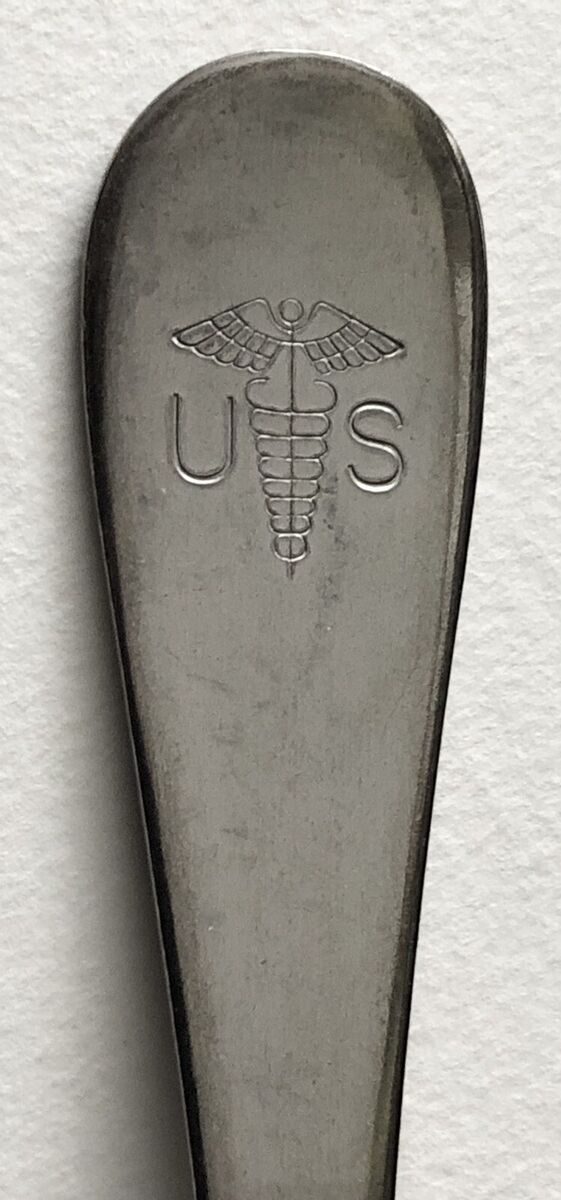The image depicts a close-up view of a stainless steel canteen fork against a white background. The polished metal object, slightly used but well-maintained, features an intricate engraving between the letters "U" and "S" at its base, depicting a figure with wings, possibly resembling a caduceus, eagle wings, or angel wings. This detailed, granite gray-colored object, leaning against a white wall with spattered designs, showcases the fine craftsmanship and utilitarian design of an Andorra setting.